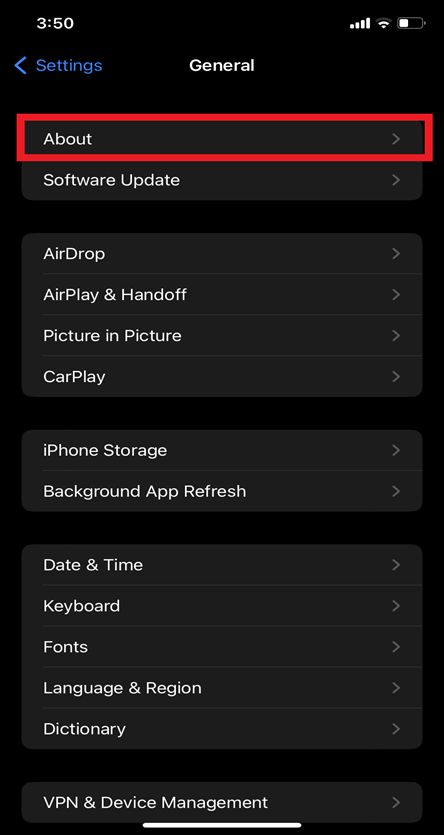A detailed screenshot of an iPhone's settings menu is displayed, notably from the 'General' section. At the top of the image, a black background with a "General" heading in large black text is visible, accompanied by a blue "Settings" option to navigate back to the previous menu. A red rectangular box highlights the "About" option, indicating it is currently selected or of particular importance. Below the "About" selection, other options are listed including "Software Update," "AirDrop," "Airplane Mode," "Handoff," "Picture in Picture," "CarPlay," "iPhone Storage," "Background App Refresh," "Date & Time," "Keyboard," "Fonts," "Language & Region," "Dictionary," and "VPN & Device Management." Each of these options features an arrow pointing to their respective sub-menus, indicating additional settings are available within each category. The iPhone's status bar is also visible, showing the battery icon, indicating remaining battery life, and the reception icon, conveying network signal strength. This detailed screenshot effectively captures the contents and layout of the iPhone's settings menu within the 'General' section.